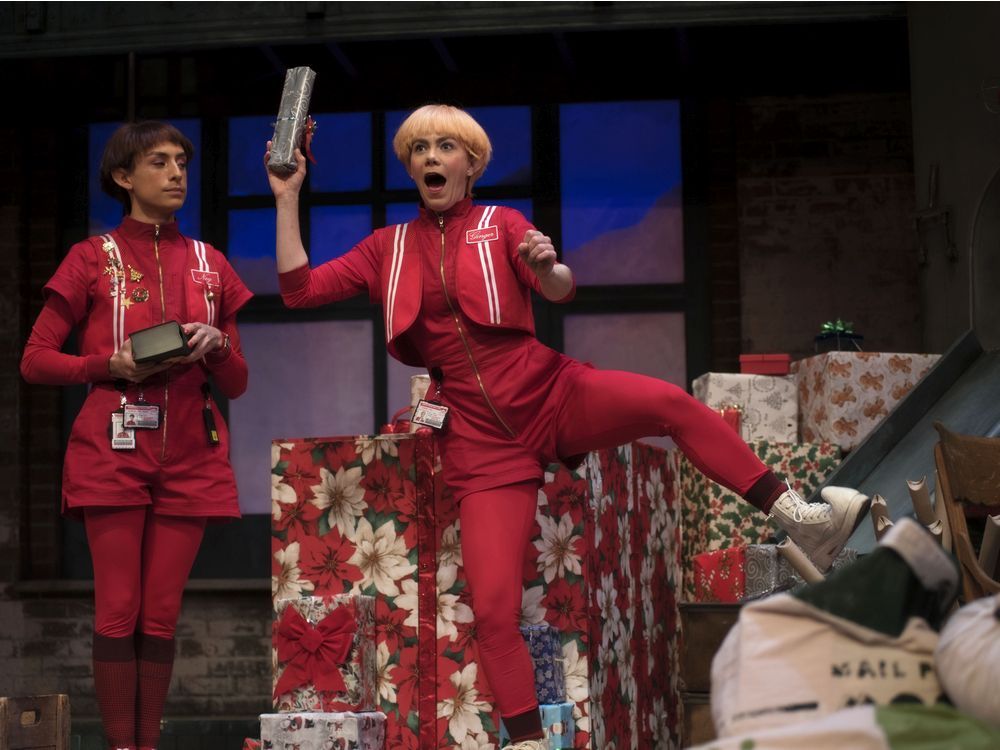This vibrant color photograph captures a lively scene from what appears to be a holiday-themed performance, likely a comedic skit or a TV show. The image features two animated women, seemingly dressed as Santa's elves. Both women don red jumpsuits with red tights, and the woman at the center, who is the focal point of the photograph, has short blonde hair. She's captured mid-jump, with her left leg extended to the side and her right arm raised, holding a gift-wrapped rectangular box. Her white shoes have curved toes, enhancing the elf-like appearance. To her left stands another woman with dark, possibly brunette, hair adorned with Christmas ornament pins on her jumpsuit. This woman is holding a gift and looking towards her blonde counterpart. 

The background showcases a festive setting with a window set in a brick wall and a plethora of Christmas presents, including a notably large gift and several smaller ones. There is also a mail bag, perhaps hinting at letters to Santa, reinforcing the holiday theme. The synthetic atmosphere and props, such as the decorative gifts and the playful mannerisms of the performers, suggest that these women are enacting a spirited and humorous portrayal of Santa's helpers.